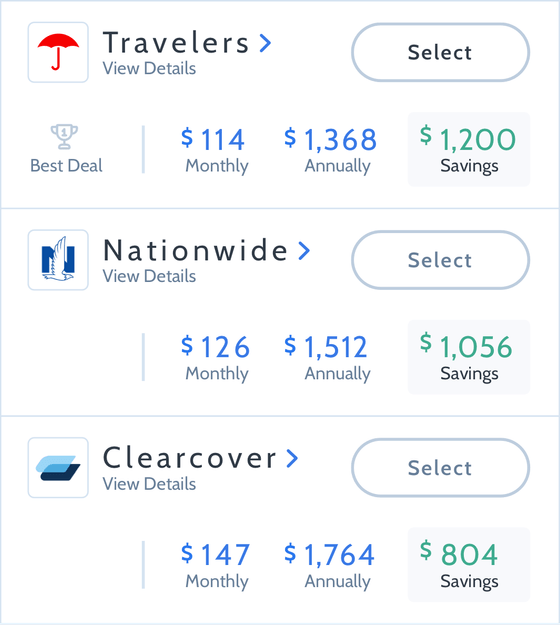The image captures a section of a screen divided into three parts, each representing different insurance options. 

1. At the top, within a highlighted rectangle, there is a red umbrella icon with the label "Travelers" next to it. Below, a "View Details" text is displayed. An arrow pointing to the right is positioned beside this text, guiding the user to the "Select" button located in the far right corner. Additionally, a trophy icon is present underneath the Travelers segment, indicating it as the "Best Deal." The pricing information shows a cost of $114 monthly, $1,368 annually, and indicates a savings of $1,200.

2. The middle section depicts the "Nationwide" option, featuring an eagle flying in front of the letter "N." Similar to the top section, it also contains a "View Details" text with a right-pointing arrow next to it and a "Select" button in the right-hand corner. The pricing for this option includes a monthly charge of $126, an annual charge of $1,512, and a savings of $1,056.

3. The bottom section represents the "Clear Cover" option. This section includes simple rectangle icons, a "Select" button on the right, and detailed cost information: $147 monthly, $1,764 annually, with a savings of $804.

This comprehensive and organized display allows users to compare the cost and savings of various insurance plans efficiently.